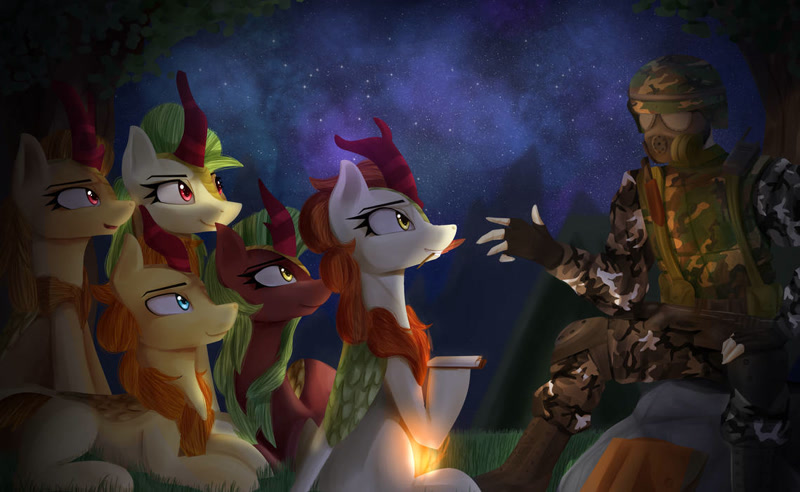In this detailed image, there is a striking piece of graphic or possibly AI-generated artwork that appears to capture a scene reminiscent of a frame from an animation or comic book. The scene is set against a stunning backdrop of a galaxy-like night sky filled with a myriad of stars in purplish and blue hues, creating a fantastically immersive atmosphere. Towards the right, a fully outfitted soldier sits on a rock. He is dressed in combat gear featuring a blend of classic and white-black camouflage, fingerless gloves showing his pale fingers, knee pads, black boots, and a gas mask that obscures his face. His attire also includes a helmet and a tactical vest, with a visible knife in a holster. A small satchel bag rests in front of him.

To his left, a group of five vibrant, humanoid horses, or ponies, gathers around, seemingly engaged by the soldier. These fantasy creatures, with large expressive eyes, exhibit a colorful palette—blending yellows, reds, greens, and browns. The white pony with a fiery red mane and yellow eyes holds a parchment and a leaf in its mouth. Nearby, a brown pony with a green mane and matching yellow eyes observes attentively. Another yellow pony, boasting blue eyes and a brown mane, lies just below them. Above it, a similarly yellow pony with a green mane and red eyes gazes at the soldier, paralleled by another yellow pony with red eyes and a faintly visible blonde mane positioned to its left.

The group sits on a patch of grass, subtly illuminated by what appears to be a campfire or lantern near the lower front part of the scene, adding to the warm, storytelling ambiance. The composition of light and shadow intensifies the contrast between the realistically depicted soldier and the fantastical elements of the ponies and the celestial background, creating a captivating and surreal narrative tableau.